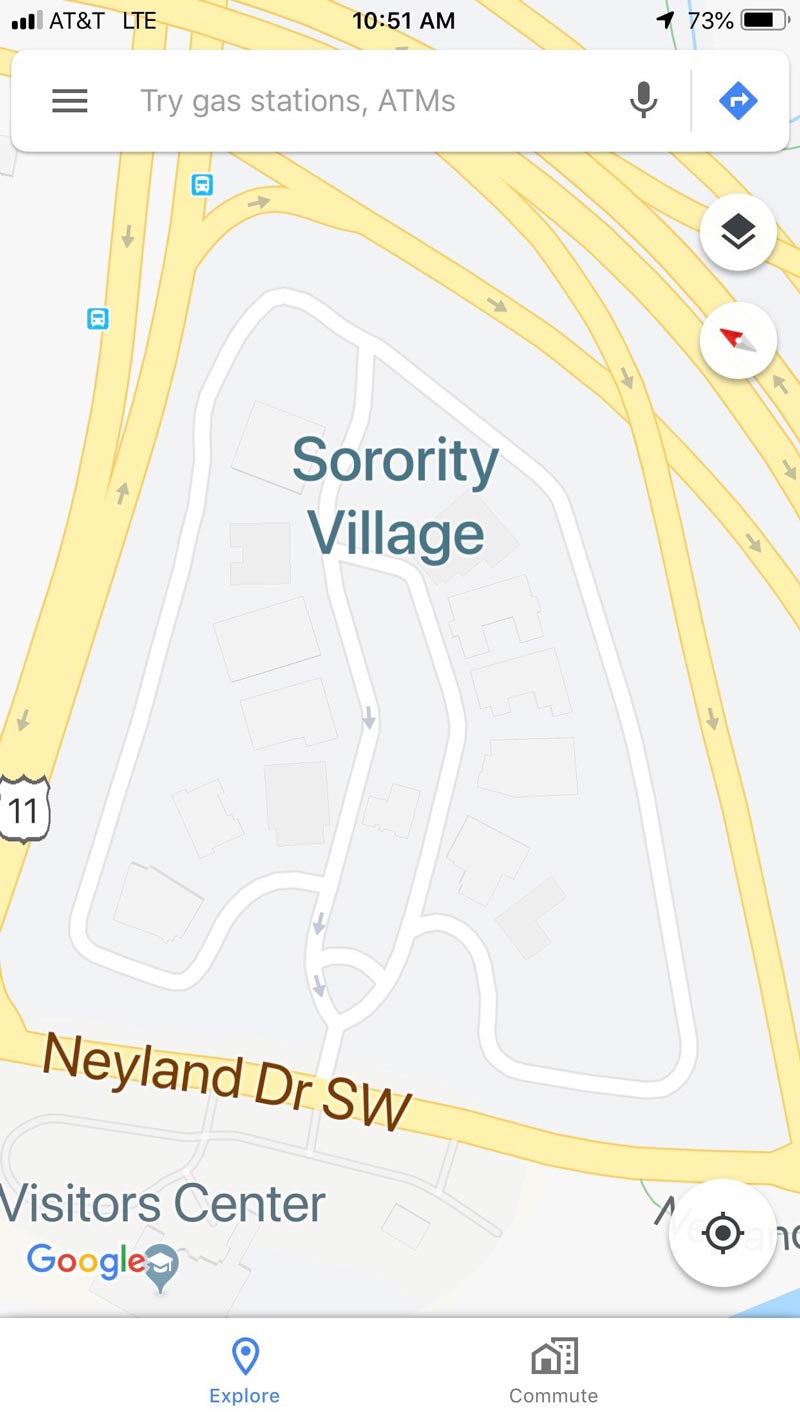A close-up view of a smartphone screen displaying a Google Maps view of a sorority village at Nayland Drive, Southwest. The screen shows a detailed map with a compass and several surrounding and intersecting roads. A floating panel above the map lists nearby TriGas stations and ATMs. The phone is connected to the AT&T network, showing the time as 10:51 AM with a battery life of 73%. The central focus of the map is the sorority village, depicted with faint outlines of inner roads and several buildings. Surrounding roads create a network that encapsulates the village area. The map provides an approximate shape of the buildings, suggesting that zooming in would reveal more detailed information.